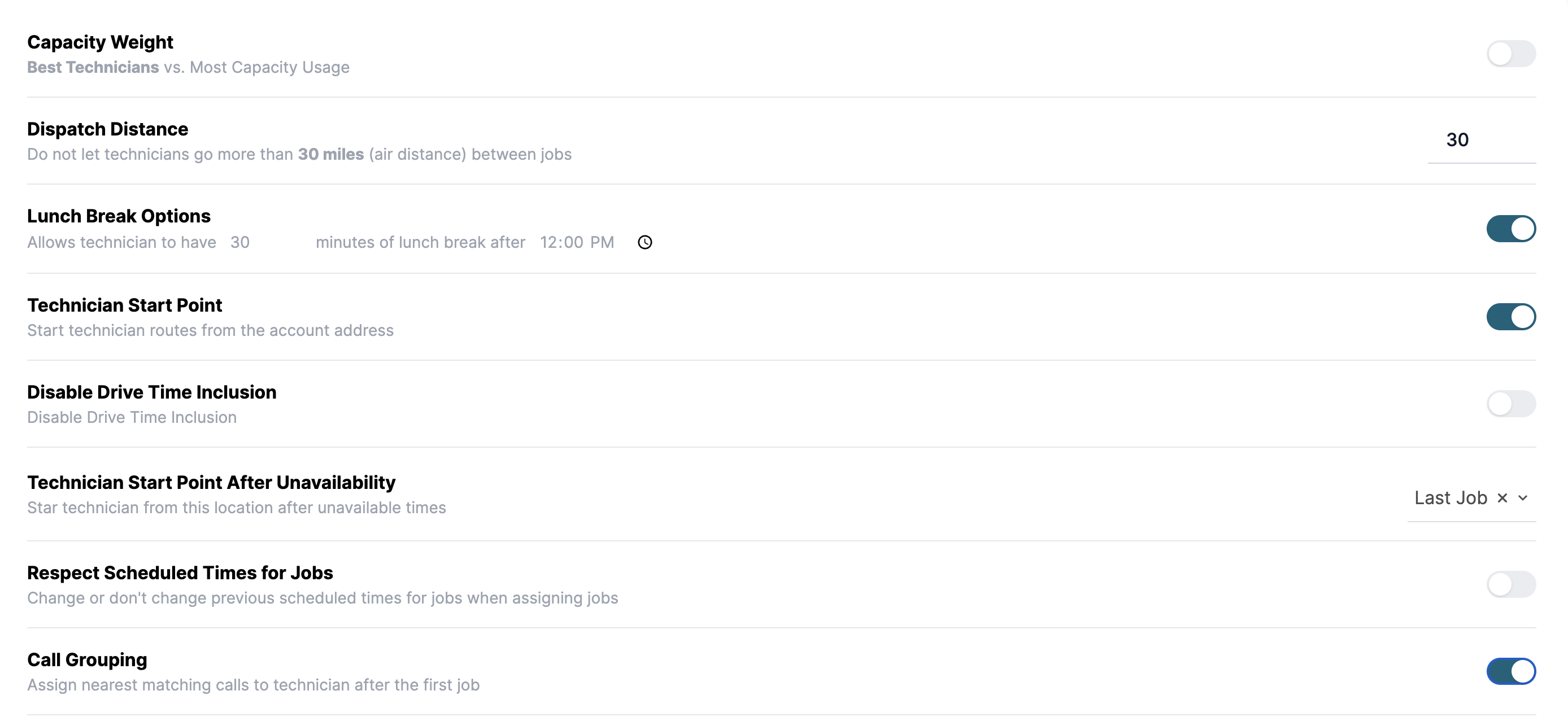**Detailed Descriptive Caption:**

The screenshot depicts a scheduling application with a clean, white background, arranged in landscape orientation. The layout consists of eight distinct rows, each delineated by a fine, faint gray horizontal line that spans the width of the page.

On the far right side of the interface, aligned along the right margin, are elongated, oblong toggle buttons designed for sliding to the left or right to activate or deactivate specific functions. The left side of the screen lists various categories, which are marked in bold text. Under each category, there is a description in regular, non-bold font. 

The first category is "Capacity Weight," with the description "Best technicians vs. most capacity usage," and it is currently not toggled on.

The second category is "Dispatch Distance," accompanied by a description that reads "Do not let technicians go more than 30 miles [something or other] distance between jobs." Instead of a toggle, this row has a customizable setting, which currently says "30," allowing users to set a specific distance.

Following is "Lunch Break Options," described as "Allows technicians to have [30] minutes of lunch break after 12 p.m." This is toggled on, suggesting it is activated.

The category "Technician Start Point" explains "Start technician routes from the account address," and this option is also toggled on.

Next is "Disabled Drive Time Inclusion," which says "Disable drive time inclusion" and is currently not toggled on.

The "Technician Start Point After Unavailability" category appears to have a typo, reading as "Star technician from this location after unavailable times" instead of "Start technician." The description says, "Last job" with a dropdown menu indicating where the technicians were last located. 

The penultimate category, "Respect Schedule Time for Jobs," advises to "Change or don't change previous schedule times for jobs when assigning jobs," and this feature is not activated.

Finally, the last category, "Call Grouping," instructs to "Assign nearest matching calls to technician after the first job," and this function is toggled on.

This completes the detailed overview of the scheduling app as shown in the screenshot.